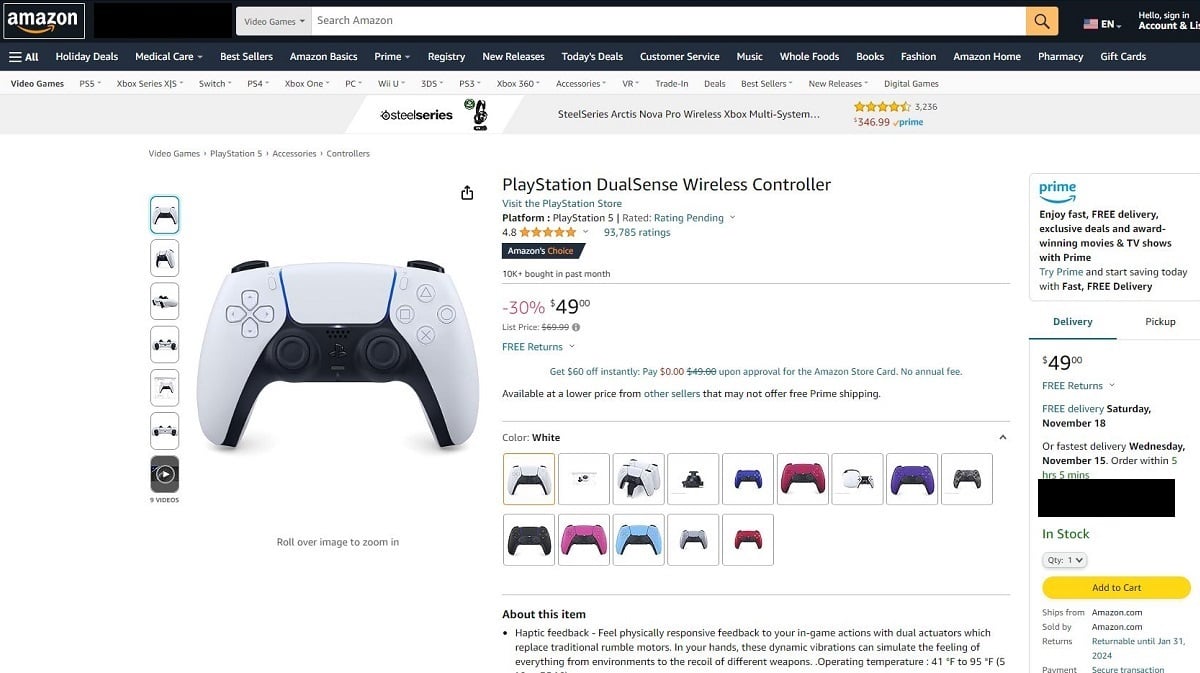On an Amazon listing webpage, the highlighted product is a PlayStation DualSense Wireless Controller, prominently featured in a sleek white and black design with blue accents. The main image showcases the controller in a front-facing view, the most traditional and recognizable advertisement perspective. The button area is primarily white, complemented by black grips and thumbsticks. To the left, different viewing angles and a video overview of the controller can be selected.

The controller is priced at $49, originally $69, reflecting a significant 30% discount. Positioned as "Amazon’s Choice," the product has an impressive 4.8-star rating derived from 93,785 customer reviews. The product, designed for use with the PlayStation 5, is available in multiple color options including hot pink, purple, light blue, gray, black, and possibly a two-pack option.

Highlighted product features include haptic feedback with dual actuators, providing responsive vibrations that simulate various in-game actions, from environmental feedback to weapon recoil sensations. Additional product details about operating temperature and a range of headers for navigating other Amazon sections like Holiday Deals, Best Sellers, and Prime offerings are also visible at the top of the page.

Customers can enjoy fast, free delivery and free returns through Amazon Prime, with delivery expected by Wednesday, November 15th. The item is in stock, and there’s a prominent yellow "Add to Cart" button displayed, emphasizing ease of purchase.